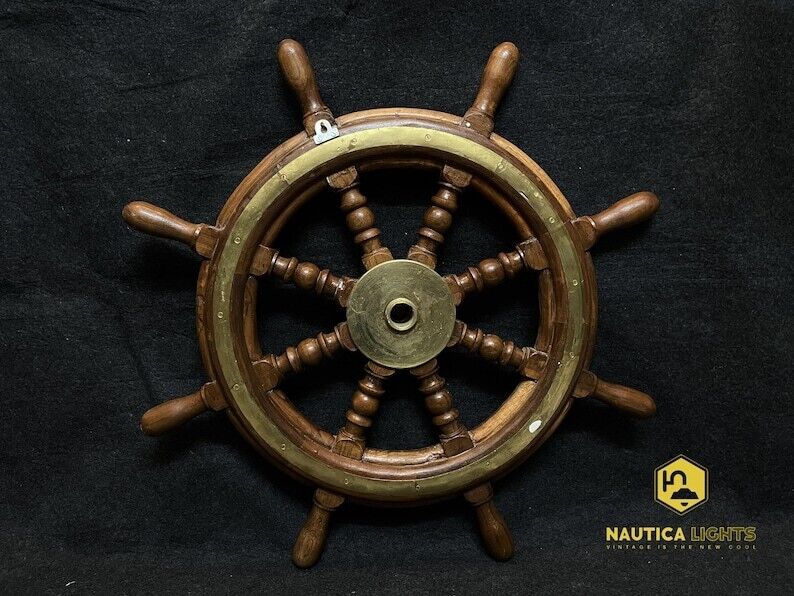The image depicts an ornate ship's steering wheel, or helm, set against a completely black background that resembles black fabric. The wheel features eight wooden spokes that extend beyond the outer rim, which is crafted from wood and adorned with a dull gold-colored metal band, brightening to a more yellow hue at the top. The spokes are intricately carved into semi-circular and square shapes, adding to the wheel’s vintage aesthetic. At the center of the wheel is another gold metal plate with a hole in the middle, through which the black background is visible. In the bottom right-hand corner of the image, there is a yellow-outlined design featuring what appears to be a lamp, possibly accompanied by a tiny boat. Below this design, the text "Nautica Lights" is visible, although a portion of the text beneath it is too small to read.